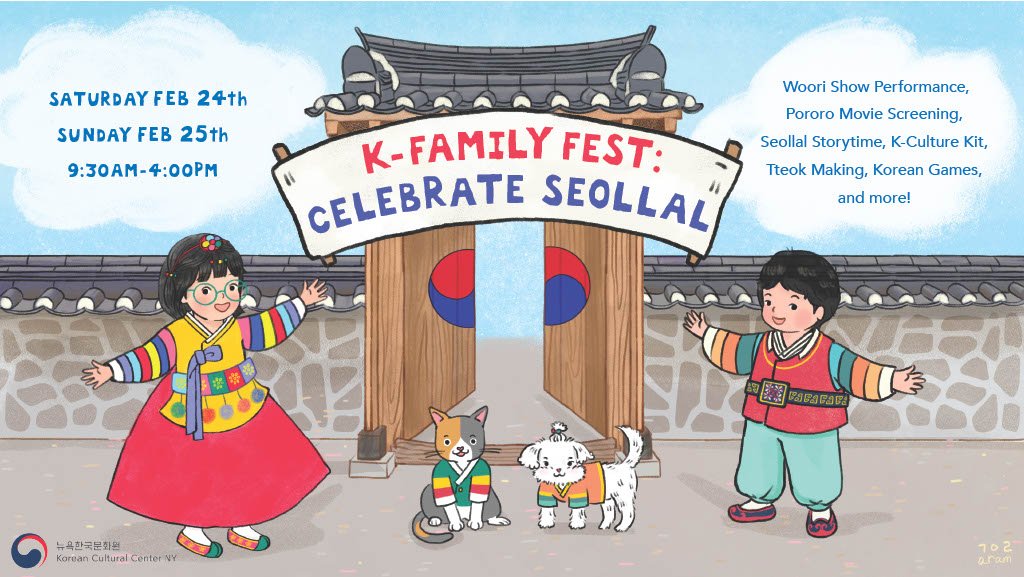The poster for K-Family Fest features a whimsical, detailed drawing set against a split background: the top half shows a blue sky with playful clouds, and the bottom half a gray, stone-like texture. Underneath an archway with a gray roof that reads "K-Family Fest, Celebrate Seollal" in a banner using red and blue colors, there are two children and two small animals. The girl, depicted in a colorful outfit, wears a pink dress with a colorful shirt on top, a bow in her short black hair, and green glasses. Next to her stands a boy in sea-green blue pants and a red shirt with a belt and colorful sleeves. Between them sit a brown, gray, and white cat and a white dog, both dressed in colorful shirts. The left-hand cloud displays the event dates, "Saturday, February 24th, Sunday, February 25th, 9:30 a.m. to 4 p.m." The right-hand cloud lists activities like "WURI Show Performance, Porori Movie Screening, Seollal Story Time, K-Culture Kit, Tteok Making, Korean Games, and more." At the bottom of the image, it says "Korean Cultural Center NY."